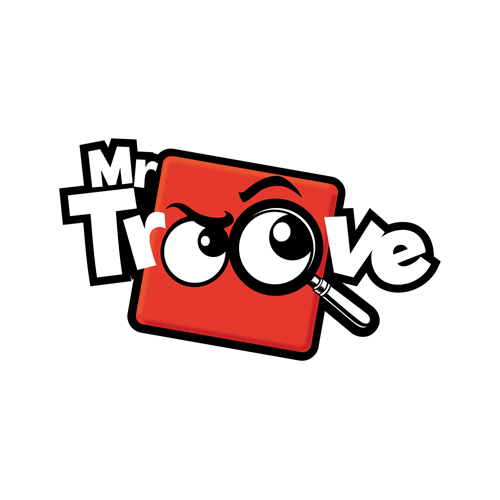The image features a cartoon-style logo on a white background. The centerpiece is an orange rectangle with a black edge, slightly turned up on the left side. Inside this rectangle are a pair of eyes with curved eyebrows, staring to the right. The eyes are depicted as circles, with the right eye magnified by a handheld magnifying glass. The text "Mr. Truth" appears prominently, with "Mr." placed above the left side of the orange rectangle and "Truth" spanning across it. The design elements suggest a detective or investigator theme, conveyed through the magnifying glass and the scrutinizing eyes. The overall color scheme includes orange, red, black, and white, with the rectangle and eyes adding a bold visual interest to the logo.